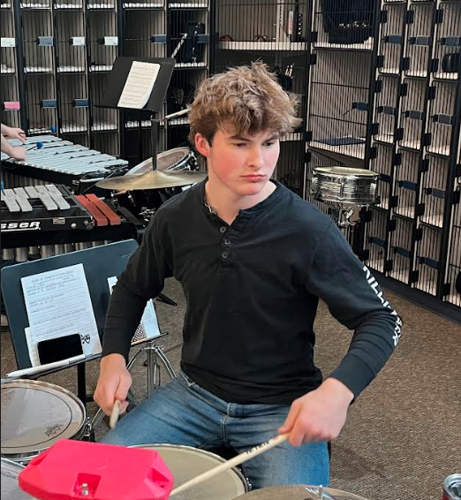The photograph, taken in portrait orientation, captures an indoor setting with a young white male, likely in his teens or early 20s, at the center. He has messy, mid-length dark blonde hair, slightly curly and appears flushed. He is dressed in a black long-sleeved top with buttons and blue jeans, and he is holding drumsticks while seated at a drum set located in the bottom left-hand corner of the picture. Only the top of the drums is visible, but there is a pinkish-red object with a protruding screw lying atop one of them. To his left, there is an easel with his cell phone and some papers.

In the background, a dull grey carpet is visible, along with other musical instruments such as a xylophone. Someone's hands are playing instruments on the left side of the frame, although the person is not visible. Additionally, there are music stands and other drum kits scattered around. The wall behind the instruments appears to be lined with cages or open-front lockers, adding to the cluttered, practice-room feel of the setting.